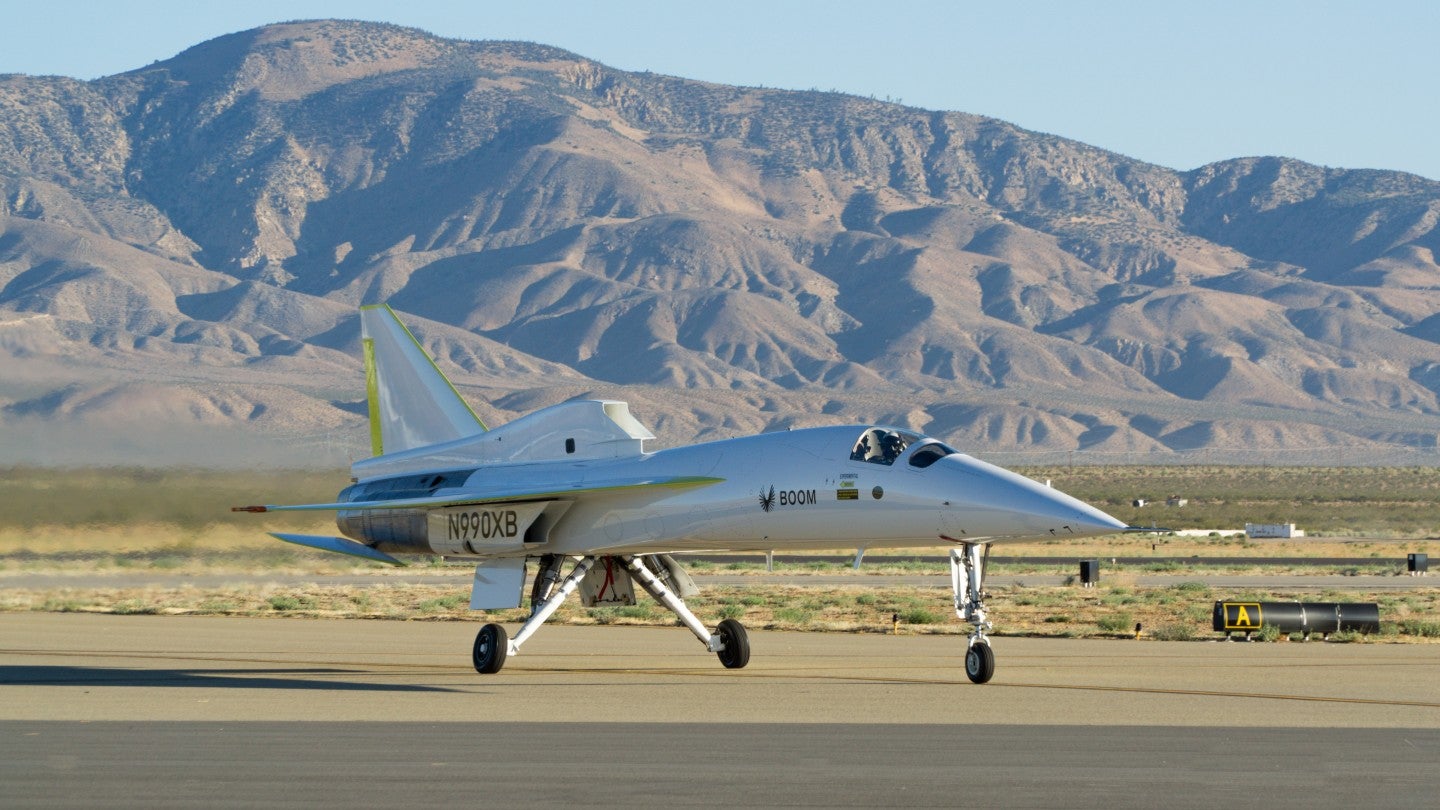The photograph captures an experimental jet aircraft taking off from a brownish runway situated in an arid, desert-like environment. The jet, which features spindly, tall landing gear with small black wheels, is white with a pointed nose and a compact cockpit, indicating it is a single-seater. The aircraft bears the markings "BOOM" on its fuselage and "N990XB" near its rear, close to the engine. The background reveals a vast, barren landscape with sparse yellow grass and a rugged, largely vegetation-free hillside under a clear blue sky, reminiscent of desert bases in California and Nevada, possibly even a secretive aerospace testing area.